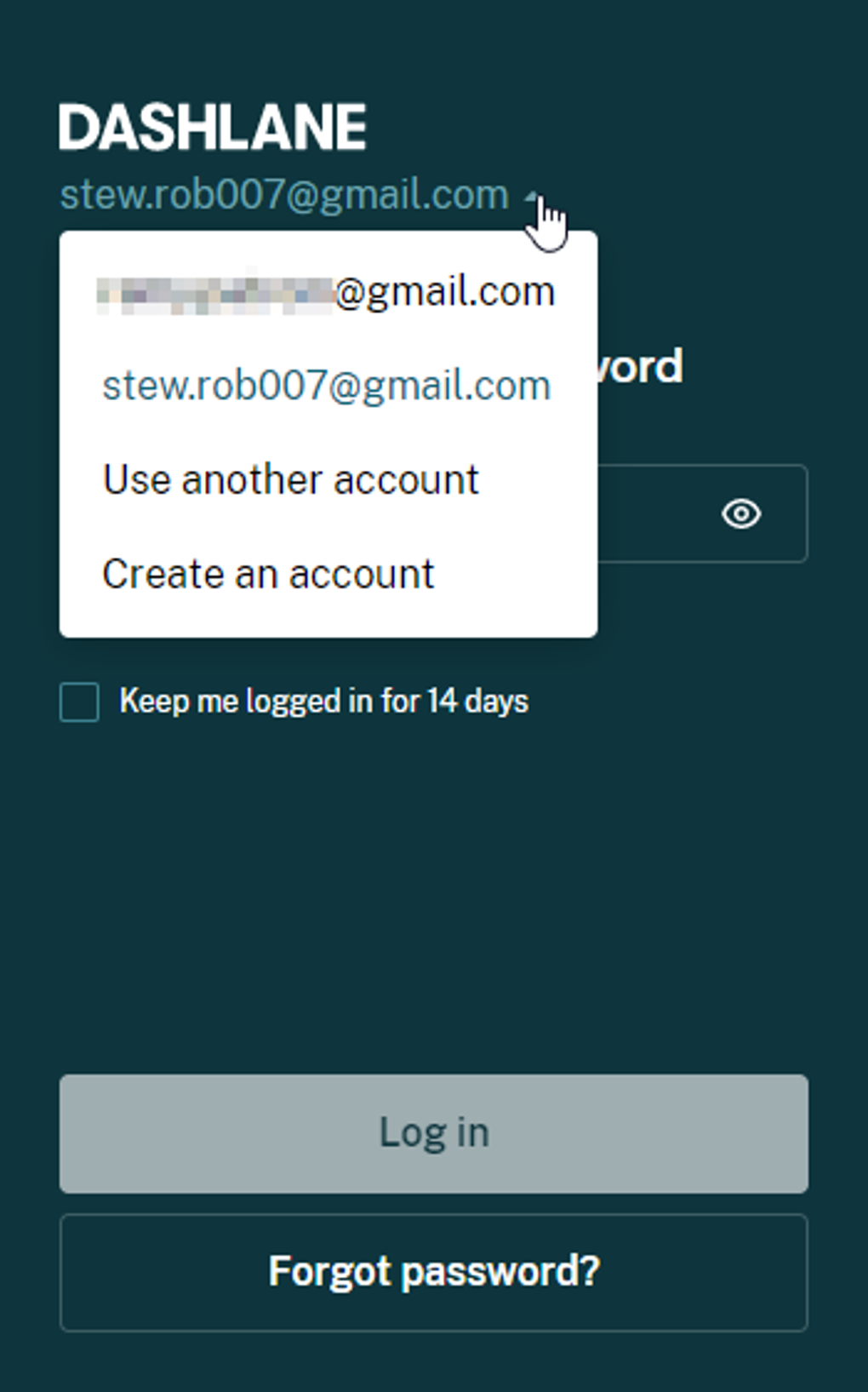The image showcases a login screen for the password manager app, Dashlane. The interface prominently displays a section for entering login details, with two Gmail accounts listed: one obscured for privacy and the other explicitly shown as stew.rob007@gmail.com. Beneath the account selection area are options to use another account or create a new one. A checkbox labeled "Keep me logged in for 14 days" allows for prolonged access, and underneath are two buttons: a gray "Log In" button and a "Forgot Password" button. The screen, minimalistic in design, features a dark blue background with white text for visibility and functionality. Additionally, there's an option to view the password being typed, a useful feature for ensuring accuracy. The irony of needing to remember the master password to access a password manager is subtly highlighted.